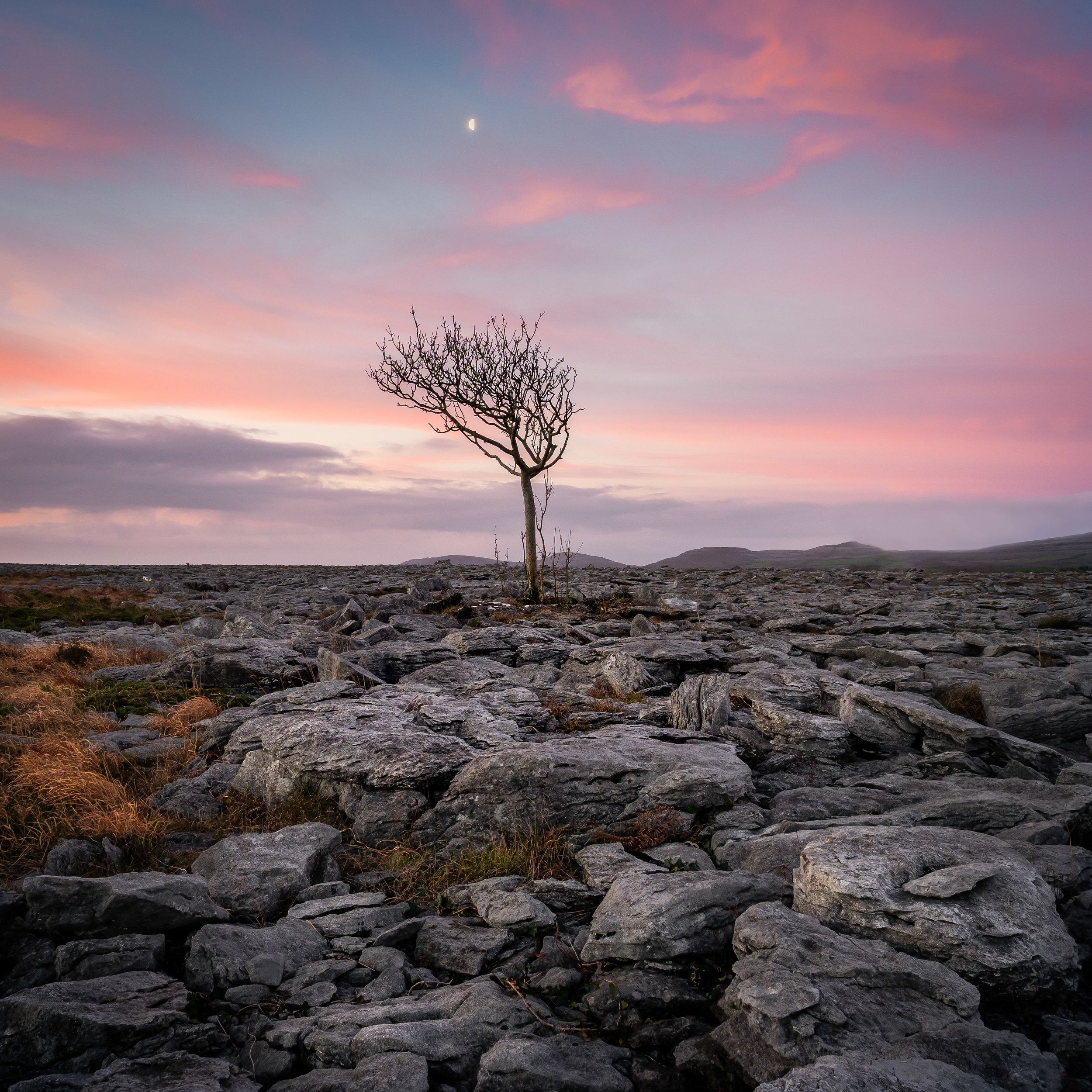In this striking outdoor color photograph, taken at sunset on a rocky, desolate landscape, a lone, leafless tree stands at the center. The tree, with its scraggly, thin, vertical branches, is surrounded by a sea of dark gray boulders and rocky terrain that stretches as far as the eye can see. Scattered among the rocks are patches of sparse vegetation, including slightly greenish but mostly orangish tufts poking through and some green moss on the left. The sky above transitions from its daytime blue to shades of pink, orange, and purple, with clouds tinged with a pink hue. Directly above the solitary tree, a bright, white half-moon hangs in the sky, casting a serene light on the scene. In the far distance, a faint mountain range can be seen, completing this vivid landscape nature photograph.